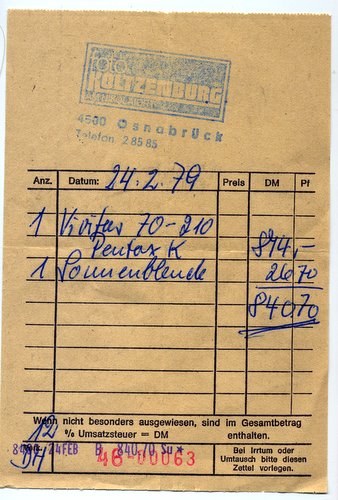The image is a portrait-style photograph of an old, light brown document, possibly a receipt or journal, with various details in German. At the top, there is a faded blue stamp that reads "Photo Koltzenberg" and below it, a clearer stamp saying "4500 S. O. Snabrook Teleton 28585" in blue. The paper features a black table with five columns labeled "ANS," "DATUM," "PRELS," "DM," and "PF," with the number "24279" written in denim blue ink. The document has handwritten cursive blue text in German that spans three lines and is difficult to read. There is also a stamped date reading "24 FEB" and what appears to be a signature or initial in blue ink on the left. The overall appearance of the document is aged, with a tan-colored background and multiple sections of printed and handwritten German text.